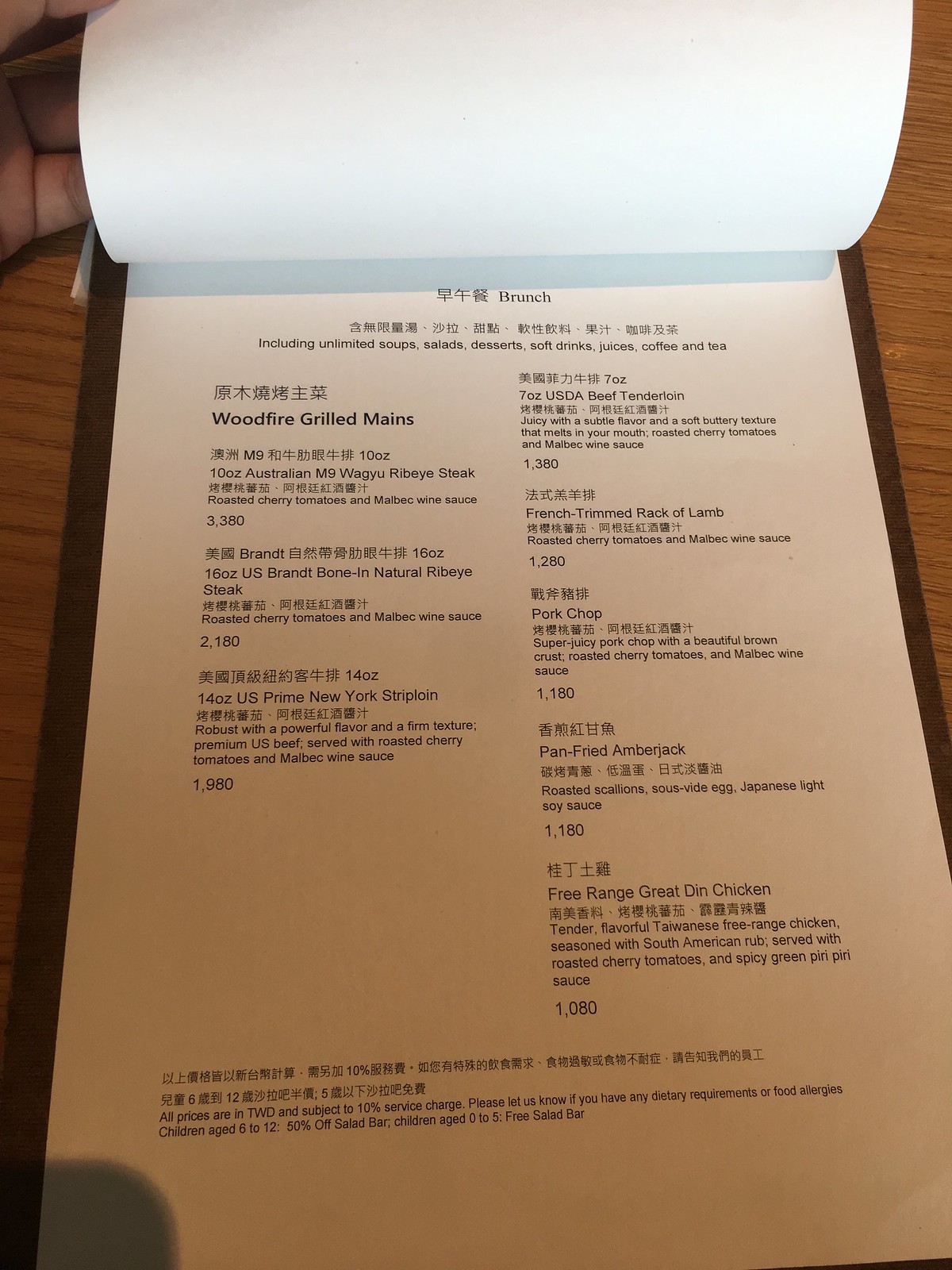The image showcases a portrait-oriented brunch menu. This bilingual menu, written in both Cantonese and English, highlights an all-inclusive brunch experience featuring unlimited soups, salads, desserts, soft drinks, juices, coffee, and tea. The top of the menu prominently displays the offerings under the umbrella title of "Brunch."

The menu is neatly divided into two columns. The left column features an array of wood-fired grilled mains, starting with an Australian Wagyu ribeye steak. Following that is a 16-ounce Brant bone-in natural ribeye steak, and then a 14-ounce prime New York strip loin. 

On the right-hand column, the delectable options continue with a 7-ounce beef tenderloin. This is followed by a French-crowned rack of lamb, a pork chop, a pan-fried amberjack, and lastly, a dish of free-range Great Gin chicken. The detailed descriptions and luxurious choices underscore a premium dining experience.